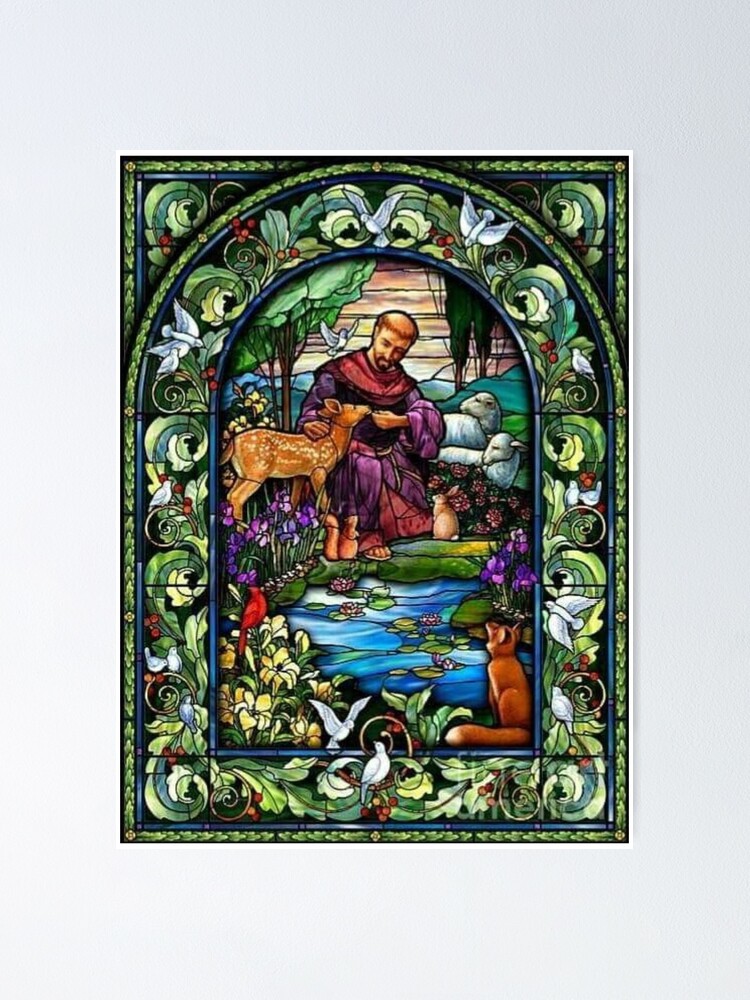The image depicts a detailed and intricate stained glass-style painting set against a light bluish-grey background, presenting an outdoor scene framed by a mosaic of green leaves, vines with white doves, red holly berries, and various vibrant flowers in shades of yellow, purple, and red. At the center of the piece, within an archway adorned with twirling leaves and berries, sits a partially bald man dressed in a red cloak with purple sleeves and tunic, accented by a moth-like collar. He is seated on rocks by a serene pond filled with lily pads and a turtle. The man is tenderly feeding a little brown deer, while around him, a gathering of animals including a fox, a turtle, a red bird, a rabbit, two lambs, and a cluster of doves can be seen. The background is painted in a warm orange hue, suggestive of a setting sun, adding a tranquil and enchanting atmosphere to the scene.